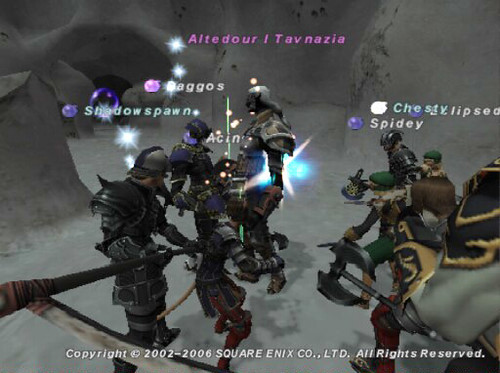The image is a screenshot from a video game, likely developed by Square Enix, as indicated by the text at the bottom of the screen: "Copyright © 2002-2006 Square Enix Co., Ltd. All rights reserved." The scene takes place in what appears to be a cavern or cave, rendered in a third-person perspective. 

In the center of the image stands a taller, armored figure named "Altedor Taznavia," as indicated by the name tag hovering above their head. They are surrounded by seven other avatars, each adorned in various types of armor and bearing different weapons. To the left, one character can be seen wielding a sword, while on the right, another character grasps a formidable double-sided axe. Each character is equipped for battle, suggesting this is a preparation or strategy moment within the game.

The detailed depiction of the characters and the immersive environment point to a high level of detail typical of Square Enix games from that era. The arrangement and gear of the avatars suggest a role-playing game where teamwork and character specialization are key elements.